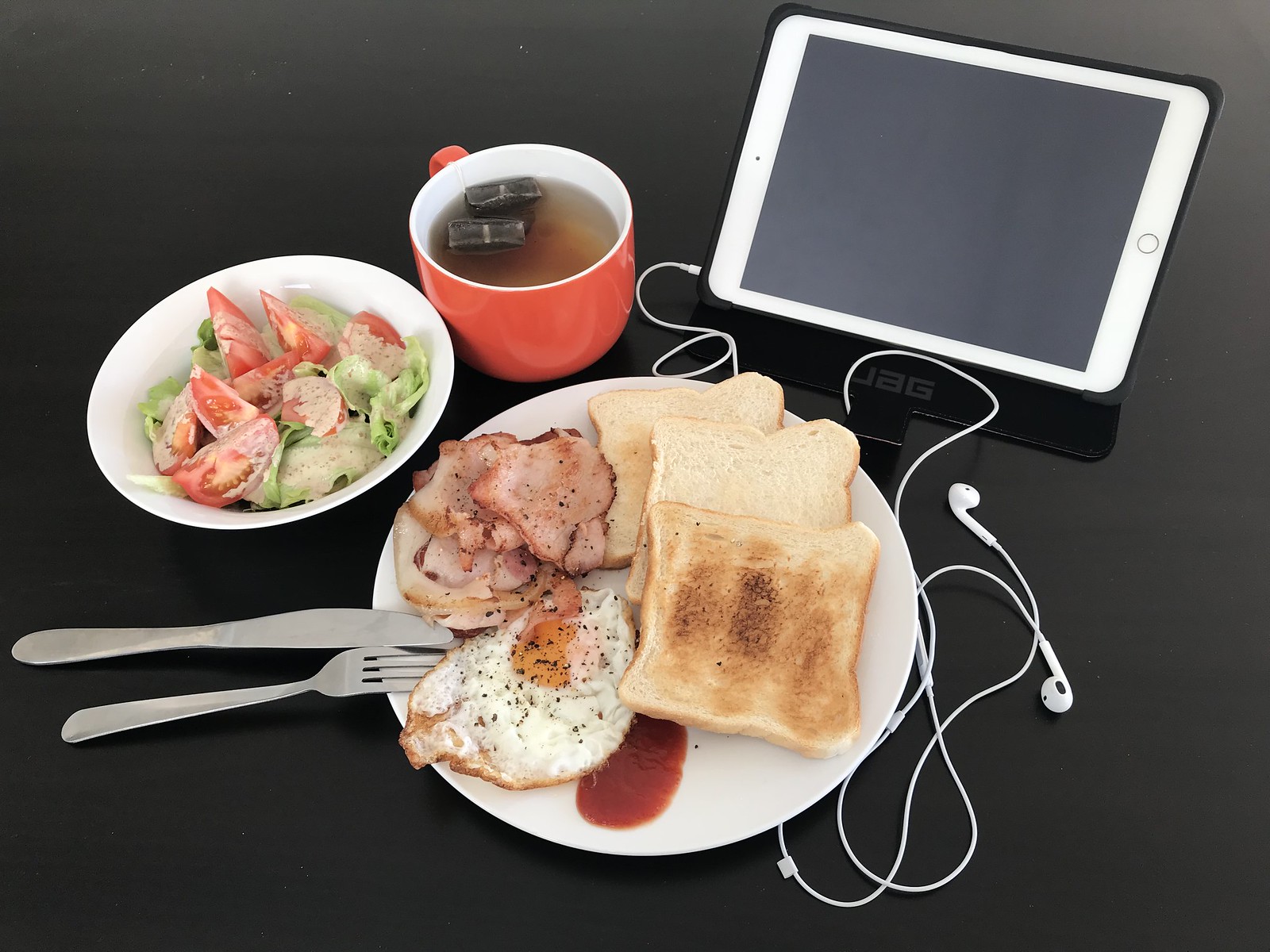In this detailed color photograph, a rectangular table setting is presented against a sleek, dark gray background. Dominating the center is a white circular plate. On the plate, starting just below a silver fork and knife resting on its left edge, there's a perfectly fried sunny-side-up egg generously sprinkled with black pepper. Next to the egg, at the bottom center of the plate, is a small serving of red sauce. Positioned at about nine o'clock, some sliced, cooked ham is arranged above the knife. Meanwhile, three pieces of lightly toasted bread occupy the right side of the plate.

To the upper left of the plate sits a white bowl filled with a fresh salad consisting of green lettuce and juicy red tomato wedges, all drizzled with a light grayish dressing. Rising above the plate at the eleven o'clock position is a vibrant red mug with a white interior, containing hot tea and two teabags with a clear liquid turning brown.

In the upper right corner of the image, an iPad in a black case stands upright. White corded earbuds extend from the iPad, resting near the edge of the plate. The overall table setup encapsulates a well-organized breakfast scene, balanced with both classic and modern elements.